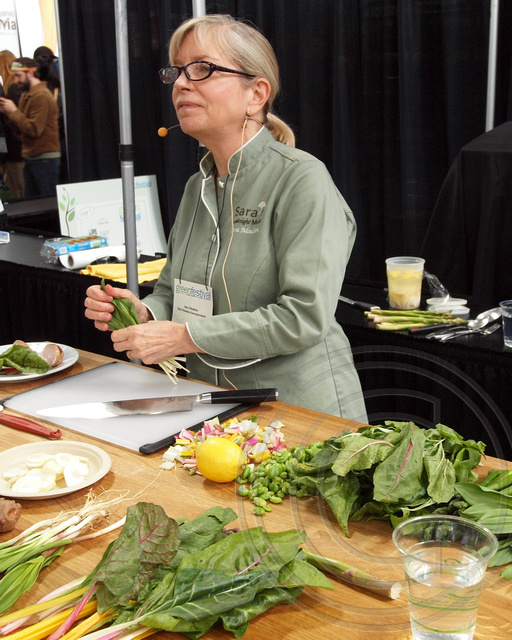In the image, a horizontally oriented photograph showcases a possible cooking show set featuring a woman in the foreground and some background elements indicative of a production environment. The woman, who appears to be Caucasian with dyed blonde hair pulled back in a low ponytail, is donned in a light green chef's jacket with white lining. She is wearing oval-shaped black-framed glasses and a yellow wearable microphone close to her mouth, perhaps suggesting she is teaching a cooking class or participating in a culinary demonstration.

The woman is positioned in front of a table cluttered with various ingredients. She holds up some leafy greens, possibly leeks or charred greens, above a white cutting board that sits prominently on the table. The cutting board also features a black-handled knife placed diagonally, alongside a lemon, chopped produce including pink and yellow chunks likely vegetables, and green leaves with pink veins. Near the cutting board, there is also a small round plastic container with a yellow substance, and scallions scattered nearby.

In the background, a black cloth curtain spans most of the scene, but behind it to the left, several individuals are partially visible, including a man in a brown sweatshirt wearing a cap pulled low over his eyes with a beard, who appears to be holding a cell phone. Various other elements such as a white panel with a tree design, a blue and white box with a yellow border, and a vertical pole enhance the complexity of the scene. Overall, the photograph blends culinary activity with behind-the-scenes details, providing a rich and dynamic snapshot of a cooking demonstration environment.